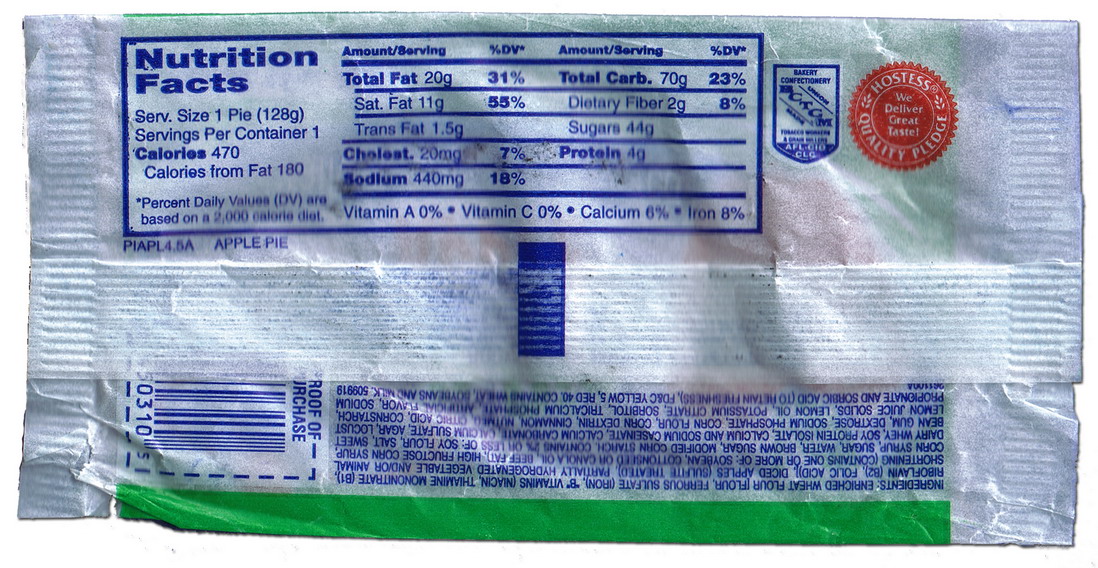This indoor close-up color photograph shows the back of a Hostess apple pie wrapper, prominently featuring detailed packaging elements. The wrapper, which is made of plastic, is mainly white with blue text and accents. The upper half of the wrapper showcases a traditional white rectangular nutrition facts label with a blue outline, detailing serving size, calories, total fat, cholesterol, sodium, total carbs, proteins, and dietary fibers, sugars, among other nutritional information. Adjacent to this label is a bakery certification shield, white, and outlined in blue, followed by a red circle with white text that reads "Hostess Quality Pledge: We deliver great taste." The center of the image is dominated by a horizontal fold line that partially obscures the print and information on the lower half of the wrapper. The bottom section includes part of a barcode and an upside-down list of the ingredients. The lowest edge of the wrapper features a thin blue (or possibly green) rectangular strip, adding to the definitive color scheme of the package.